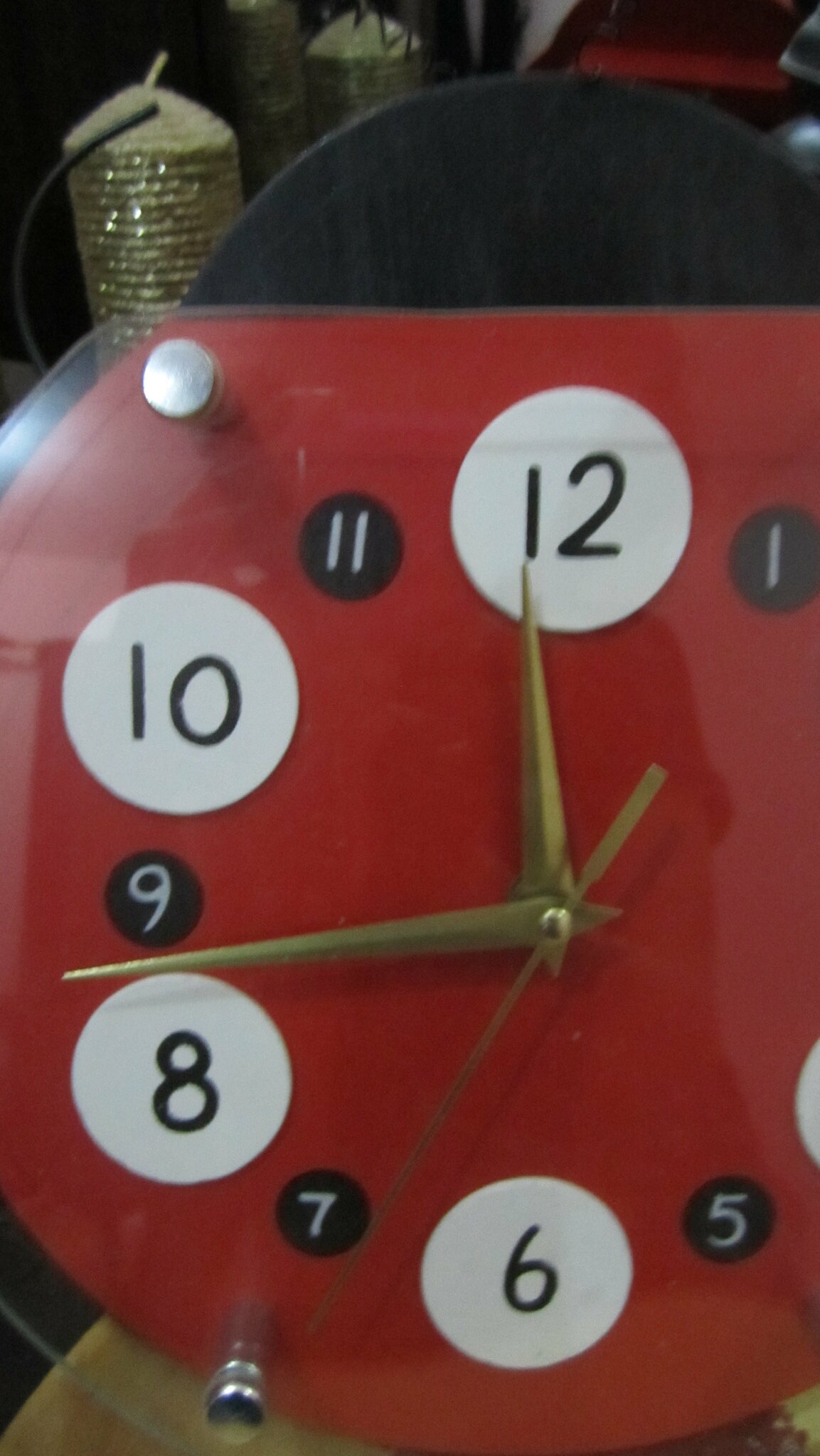This image features a vibrant red clock designed to resemble a ladybug. The clock has a distinct black hump at the top, adding to its charming ladybug appearance. The clock face displays the numbers 12, 6, 8, and 10 prominently, each encased in large white circles. In contrast, the numbers 1, 5, 7, 9, and 11 are smaller and set within small black circles. The larger numbers are black, while the smaller ones are white.

The clock has three hands: a short one indicating the hour, pointing at the number 12; a medium-length, skinny hand marking the minutes, positioned between the numbers 8 and 9; and a long, thin second hand directed between the numbers 6 and 7. The clock face is protected by a clear material secured with silver metal rivets.

In the background on the top left, there is a concrete post with a black hose attached, adding an industrial element to the vivid and whimsical scene.